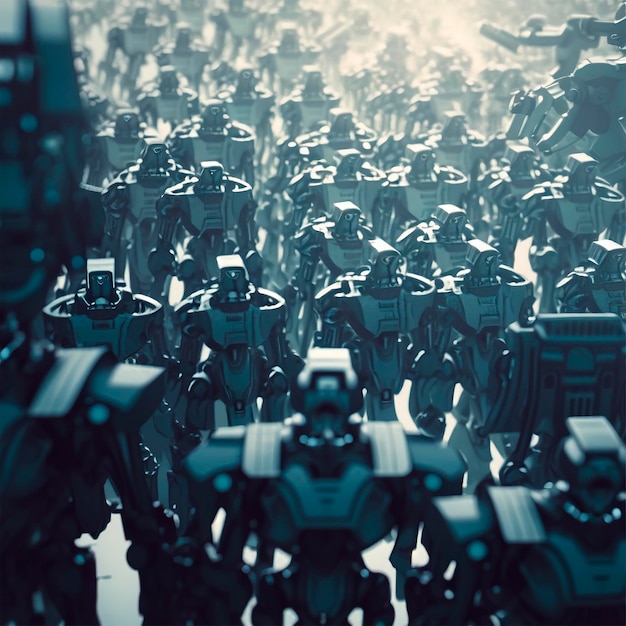The image is a digitally created rendering showcasing an army of robots, uniformly lined up and facing the camera. Each robot features a large metal body with broad shoulders, a square head with a singular, round eye, and a prominent jaw-like structure. They appear to be clad in bulky armor, enhancing their mechanical and imposing presence. The robots are bluish-gray, with some white highlights suggesting light reflections. In the foreground, three robots are visible, although somewhat out of focus and blurry. Behind them, rows upon rows of similar robots extend into the background, becoming progressively more indistinct and blurry. This formation hints at countless identical robots marching in unison, emphasizing the sheer scale of the depicted robotic army.